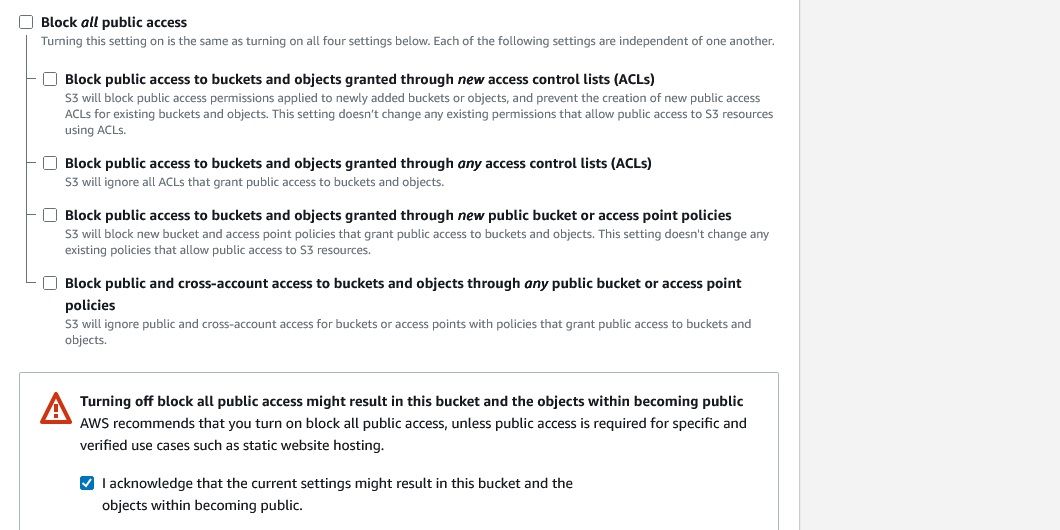In this image, there is a detailed interface for managing public access settings for a particular site. Central to the image is a prominent, white square box. Adjacent to this box, the text "Block all public access" is displayed in bold, black letters. Beneath the header, a descriptive explanation is provided.

From the white box, a straight line extends vertically downward, traversing through four segmented lines until it reaches another box. This secondary box encloses four smaller sub-boxes, each representing a distinct access option.

1. The first sub-box is labeled "Public access to buckets and objects granted through new access control lists (ACLs)."
2. The second sub-box is titled "Block public access to buckets and objects granted through any access control lists (ACLs)."
3. The third sub-box states "Block public access to buckets and objects granted through new public bucket or access point policies."
4. The fourth and final sub-box reads "Block public and cross-account access to buckets and objects granted through any public bucket or access point policies."

Below these options, a warning message is present: "Turning off block all public access might result in this bucket and the objects within becoming public."